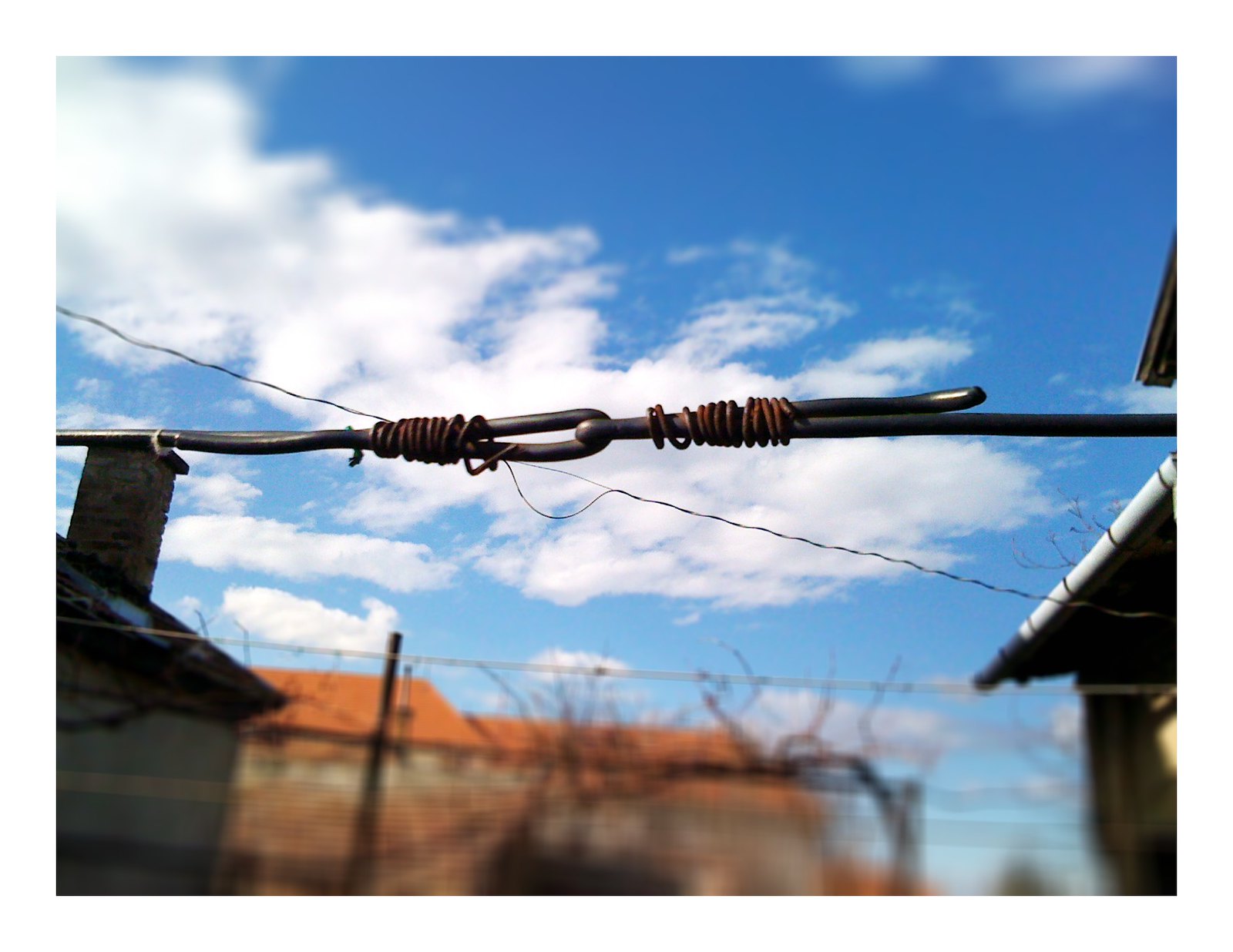The image captures a detailed, close-up view of two intersecting metal cables, one wrapping around the other with small metal wires securing the connection. The background features a neighborhood scene with a mix of houses and possibly apartment complexes. Prominent in the scene is a house on the right, showing a gutter and an upper dormer, and a house on the left with a brick chimney. There's a red-roofed building further back. The photograph is taken in broad daylight, under a blue sky adorned with fluffy clouds, which deepen in color towards the top of the image. While the central focus of the image remains sharp, it becomes blurry towards the bottom, adding to the dynamic quality of the photo. The scene is devoid of people and vehicles, emphasizing the tranquil, everyday nature of the setting.